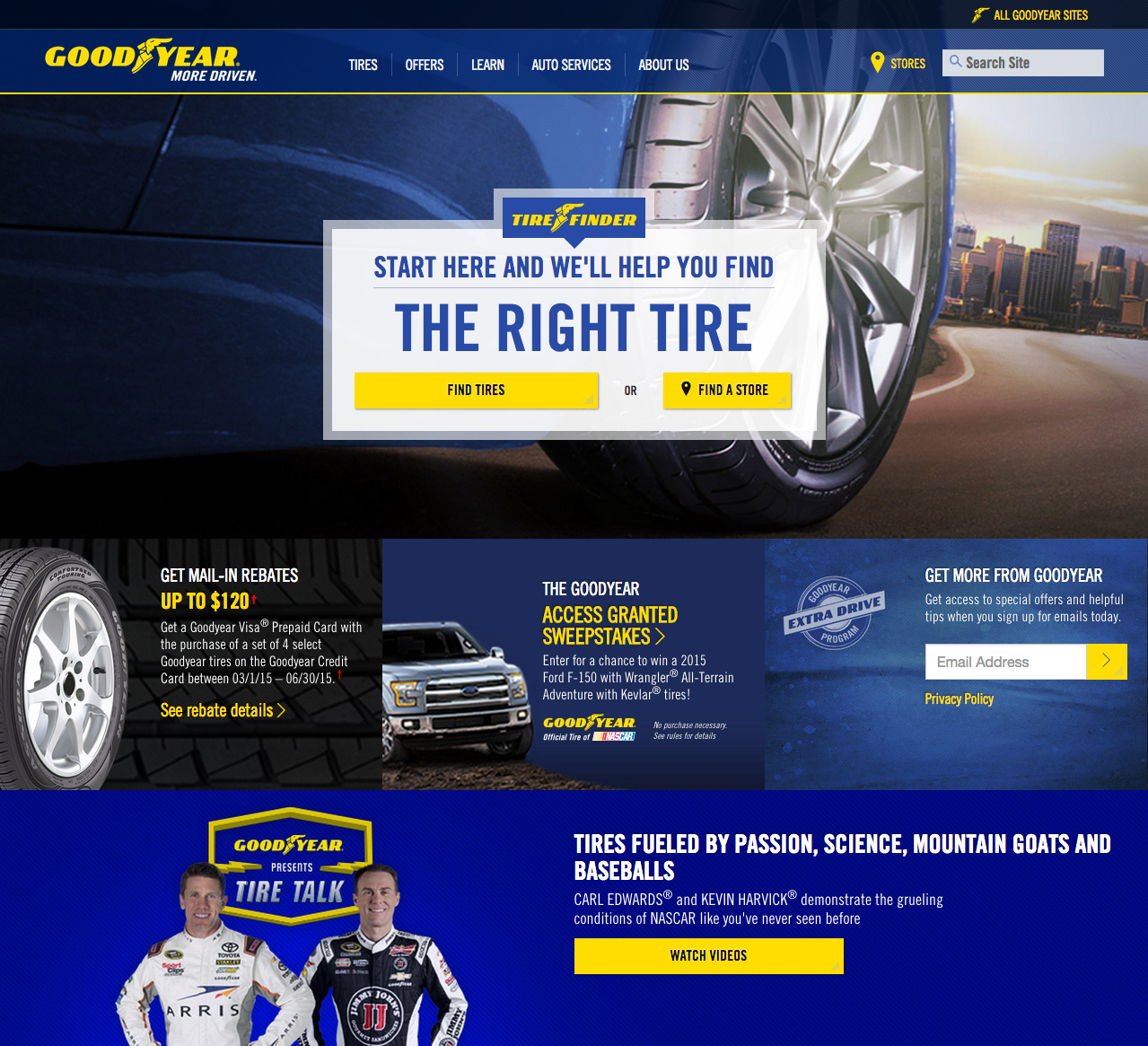This image captures the homepage of the Goodyear website. Prominently featured at the top are navigational links, including "Tires," "Offers," "Learn," "Auto Services," "About Us," "Stores," and a "Search Sites" bar. The center of the page highlights the "Tire Finder" tool with a prompt stating, "Start here and we'll help you find the right tire," along with options to "Find Tires" or "Find a Store." A banner promotes mail-in rebates and the Goodyear Access Granted Sweepstakes, offering a chance to win a 2015 Ford F-150 equipped with Wrangler All-Terrain Adventure with Kevlar tires. Additional sections encourage visitors to get more from Goodyear by signing up for emails, which provide access to special offers and helpful tips. The page also features a slogan, "Tires fueled by passion, science, mountain goats, and baseballs," and invites users to watch videos related to Goodyear products and services.